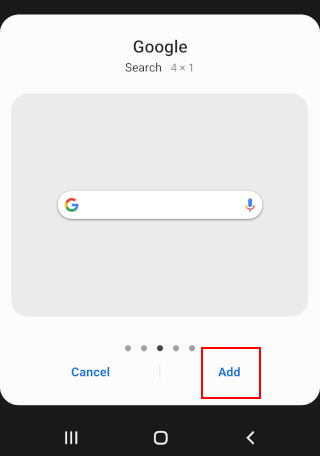The image features a minimalist design with a stark white background. Dominating the top part of the image is a thick, black line, while the bottom part is anchored by a large, heavy black box. 

In the central area of the image, the word "Google" appears in blue letters, alongside a few interface elements denoted as "Search" and "4x1." There's also a prominent blue square containing a Google search box, displaying the iconic multi-colored 'G' logo in red, yellow, blue, and green. Adjacent to the 'G' logo is a small microphone icon rendered in red and blue.

Below the search box is a white rectangular area with five dots in a horizontal arrangement, the middle dot being thin and black. Two buttons are placed below this area: one blue button labeled "Cancel" and one red box labeled "Add."

Within the heavy black box at the bottom part of the image, there are three horizontal lines, a square, and a left-pointing arrow. This layout represents a Google search interface with customizable options and navigation elements.